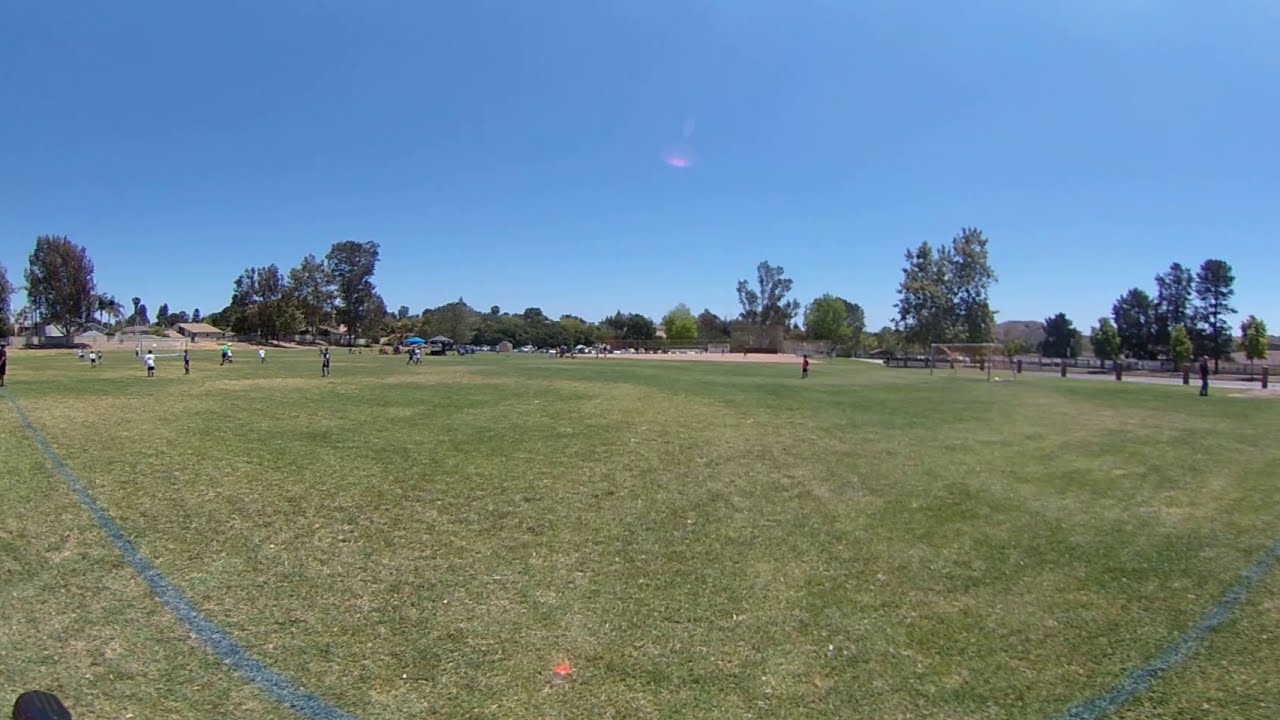This horizontally aligned, outdoor daylight photograph captures a vast sports field in a park, characterized by closely mown green grass with occasional brown patches. Blue spray-painted lines stretch across the grass, marking the field's boundaries, which seem to extend both to the right and left from the image's corners. In the foreground, the grass is unoccupied, while in the distance, small figures of people, potentially children, are visible, donned in various jersey colors, including white and dark shades. They appear to be dispersed across the field, possibly playing a sport, though the specific game is unclear from this distance. A solitary soccer goal with a net stands off to the right side of the image. Further back, the scene includes a road delineated by vehicle barriers, as well as a parking lot with several parked cars. Additionally, a couple of umbrellas, one blue and one black, are set up near the lot. On the horizon, low buildings with peaked brown roofs are partially obscured by tall trees that line the middle of the photograph. The top of the image is dominated by a clear, vibrant blue sky with a single, feathery white cloud drifting in the center.